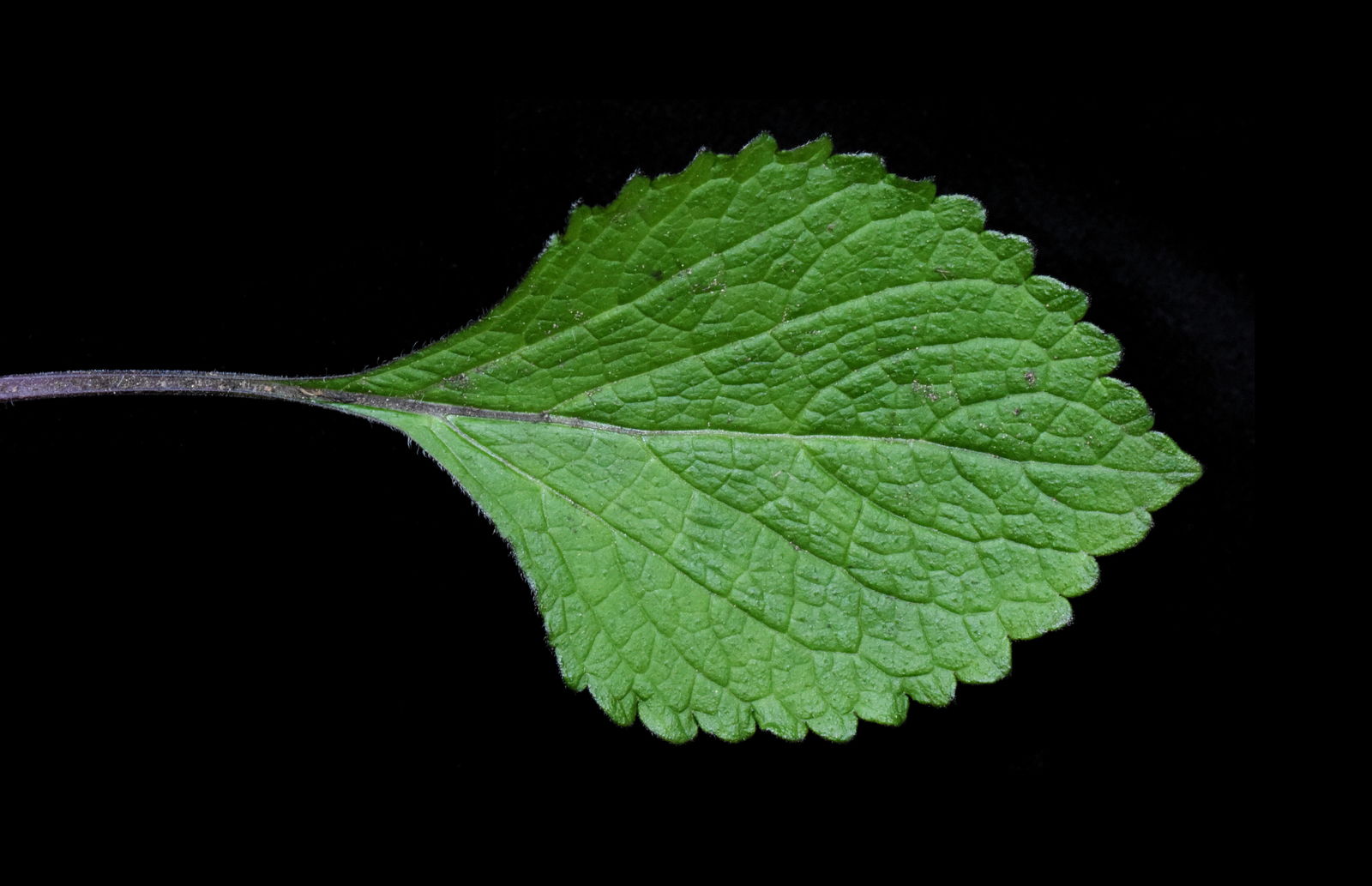Against a plain, completely black background, there is a detailed close-up image of a single green leaf. This medium green leaf, which appears textured and almost fuzzy, has an intricate design reminiscent of interlocking feathers. Its edges curve upwards, forming ridges, and it is covered in fine hairs along the borders. The leaf’s veins and spine are prominently visible, with the stem starting as a light gray color on the left side and growing darker and slightly purplish towards the center, where it merges with the leaf. The leaf points to the right, with light seemingly shining on the bottom side, enhancing the textures and details. The black backdrop emphasizes the solitary nature of this small, yet vividly captured, leaf.